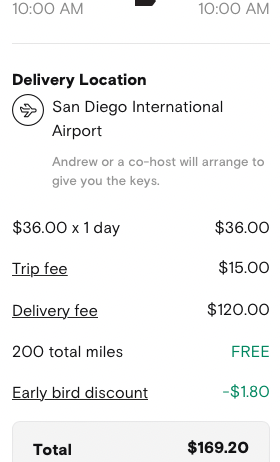Screenshot of a delivery confirmation or reservation, possibly related to an airport or Airbnb service. The top section displays a clock showing 10 a.m., indicating the time of the capture. The screenshot appears to have been taken on a smartphone. In the upper left corner, bold black text reads "Delivery Location" with an icon of a plane inside a circle next to it. The adjacent text specifies "San Diego International Airport," and mentions that "Andrew or a co-host will arrange to give you the keys."

Below this information, it lists financial details: 
- Price of $36.00 for one day
- Trip fee: $15.00 (underlined)
- Delivery fee: $120.00
- 200 total miles included for free
- Early bird discount: $1.80 (in teal font)

At the bottom, in bold black text, it states "Total," followed by the final amount of $169.20. Due to the ambiguous nature of the information and lack of branding, it’s unclear whether this is related to an Airbnb arrangement, a transportation service, or another type of delivery.